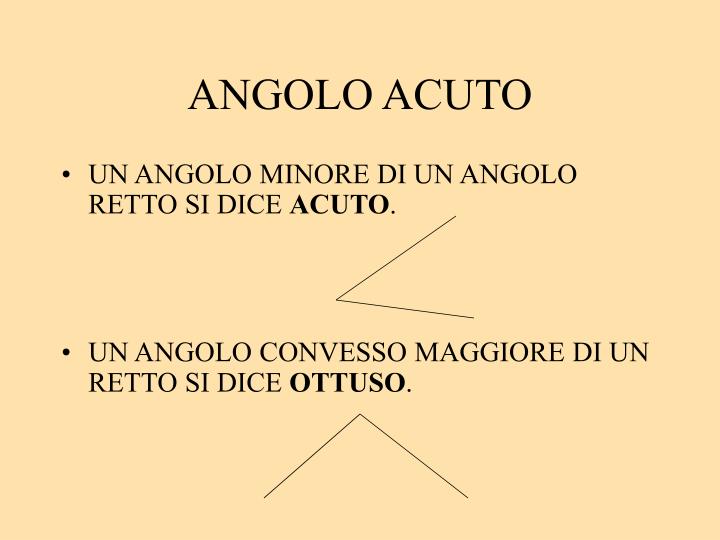The image features a horizontal, rectangular design with a yellowish beige, or tan, background resembling parchment or ivory. Dominating the content is black text presented in what looks like a typewriter font, entirely in capital letters. The text is in Italian and begins with a bold headline reading "ANGOLO ACUTO." Below, there are two bullet points. The first bullet point states, "Un angolo minore di un angolo retto si dice acuto," accompanied by a simple diagram of two black lines at an acute angle. Following this, the second bullet point reads, "Un angolo convesso maggiore di un angolo retto si dice ottuso," illustrated with another diagram of two black lines forming an obtuse angle. The infographics include clear visual aids, such as circles around the text and a couple of open triangles. Overall, the image serves an educational purpose, explaining the characteristics of acute and obtuse angles in Italian.